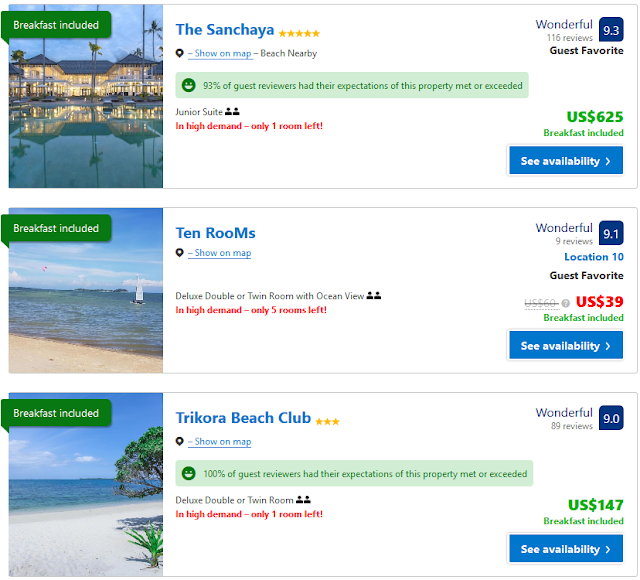### Vacation Rentals Listings

#### 1. Sanshia Waterfront Complex
A stunning vacation property built over tranquil waters, the Sanshia offers a mesmerizing view with its illuminated structures reflecting beautifully in the water at dusk. The complex includes numerous amenities with a green banner across the top of the image indicating "breakfast included." The listing proudly boasts a perfect 5-star rating, and mentions a nearby beach. Impressively, 93% of guest reviews reported exceeding their expectations. Priced at $625 per night, it’s a popular choice, highlighted by the "in high demand" notice with just one room left. The listing provides an option to check availability and shows it on the map for easy location.

#### 2. Oceanfront Sailboat View
This serene image captures a sailboat peacefully floating on pristine blue waters under a clear blue sky. It showcases a beach with no people in sight, emphasizing tranquility and exclusiveness. The listing indicates there are 10 rooms available, with specific mention of a "Deluxe Double Twin Room" offering a stunning ocean view. Priced at an affordable $39 per night, this property has received an impressive review score of 9.1 out of 10. Currently, there are only five rooms left, making it a swiftly booking choice for travelers.

#### 3. Tricora Beach Club
Showcasing a beautiful stretch of sandy beach under a cloudy sky, the Tricora Beach Club is another enticing vacation destination. Although the image does not reveal the rooms, the lush beach landscape sets an inviting tone for a beachside retreat. The property is listed at $147 per night, providing a balance of luxury and affordability. The listing includes the location on a map for convenience, ensuring guests can plan their travel with ease.